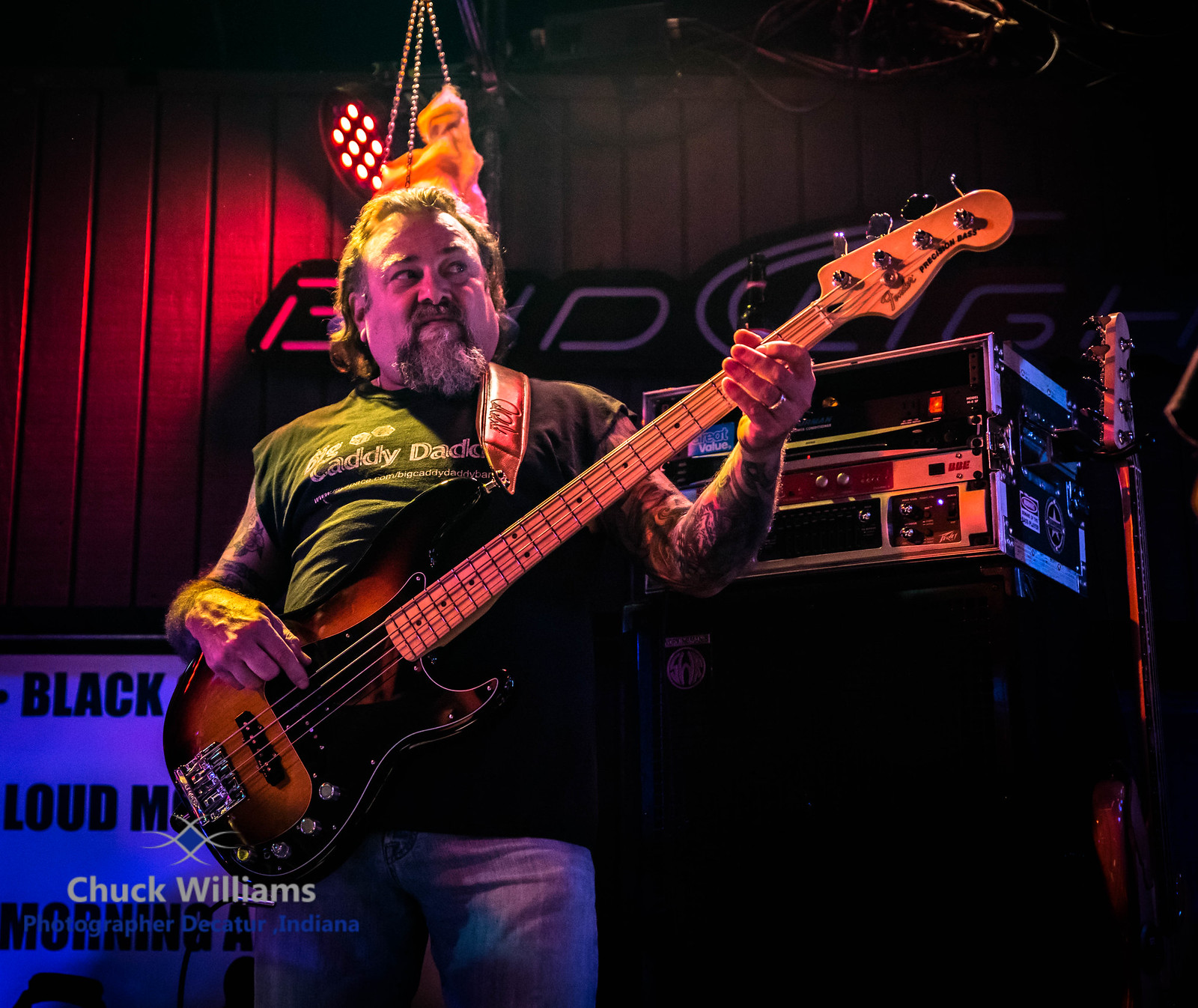In this image, a man stands on a stage illuminated by a striking red spotlight, playing a bass guitar. He has his dark hair pulled back and sports a goatee that is brown with a touch of gray. Dressed in a black sleeveless shirt emblazoned with "Catty Daddy" and blue jeans, he appears slightly overweight. Behind him, to his left, is a speaker or stereo system, and nearby, another guitar can be seen lined up. Stage lights and a Bud Light sign are visible in the background. In the lower left corner, the picture bears the inscription "Chuck Williams, photographer, Decatur, Indiana" in white font. The man's poised presence and the rich details of the stage set-up capture a vivid moment during his performance.